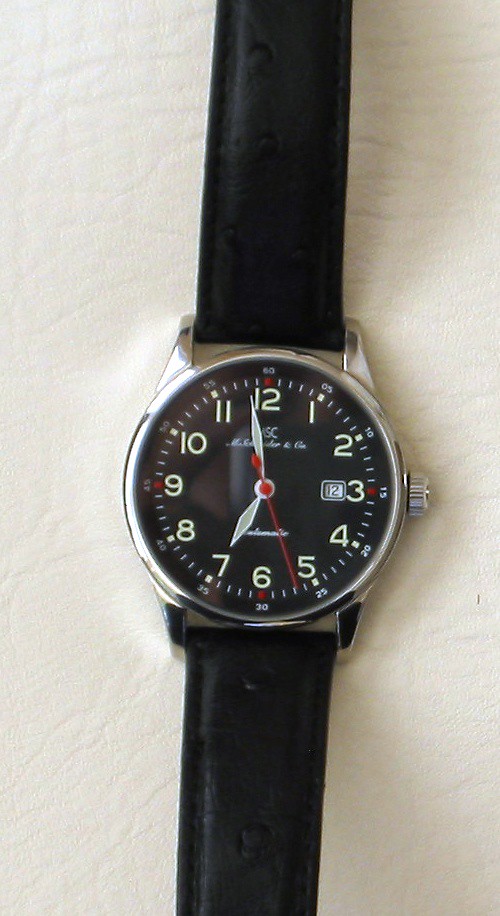This detailed, close-up photograph features a wristwatch set against a pristine white background. The watch showcases a sleek, round silver housing, complemented by black wristbands, which appear to be either faux leather or genuine leather. The inner watch face stands out with its black background and a combination of white and beige details. Specifically, the watch displays white numeric hours from 1 through 12, along with white hash marks for the seconds between them. The beige numbers and squares may contain luminescent paint, suggesting they glow in the dark. 

The precise time shown is approximately 6:57, with the hour hand pointing at 7, the minute hand near the 12, and the red second hand positioned just past the 5 toward the 6. Notably, a small square next to the 3 indicates the date, with the current date shown as 12. Additionally, a small silver dial protrudes from the right side of the watch, likely for setting the time and date. The watch’s elegant design and meticulous details are accentuated by the clear, natural lighting, hinting at either a bright morning or a long, sunny evening.